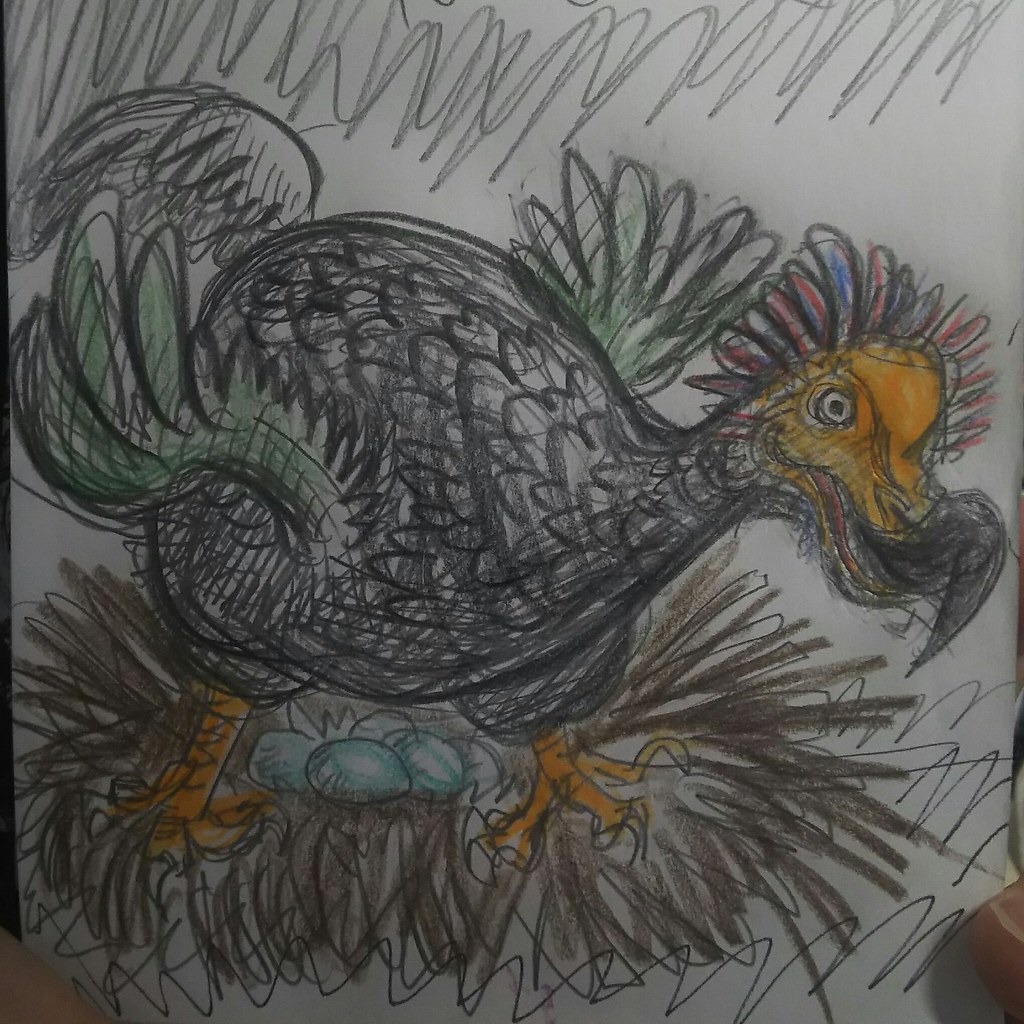A hand-drawn illustration depicts a unique bird perched on a nest filled with four small, blue eggs. The creature, reminiscent of a dodo bird or an unusually shaped chicken, sports a yellow head with a distinctive hump. A prominent feature of the bird is its large, black appendage, which could be interpreted as either a horn or an extended tongue, curving upwards and then tapering to a point. Surrounding its head and trailing down its neck are colorful, looping patterns in red and blue, adding a whimsical element to its appearance. The bird's body features two protruding green feathers, while its sturdy, orange legs with three toes each support it within the nest. The nest itself is a chaotic cluster of lines, extending downward and outward, encapsulating the eggs and providing a base for the bird's peculiar stance.